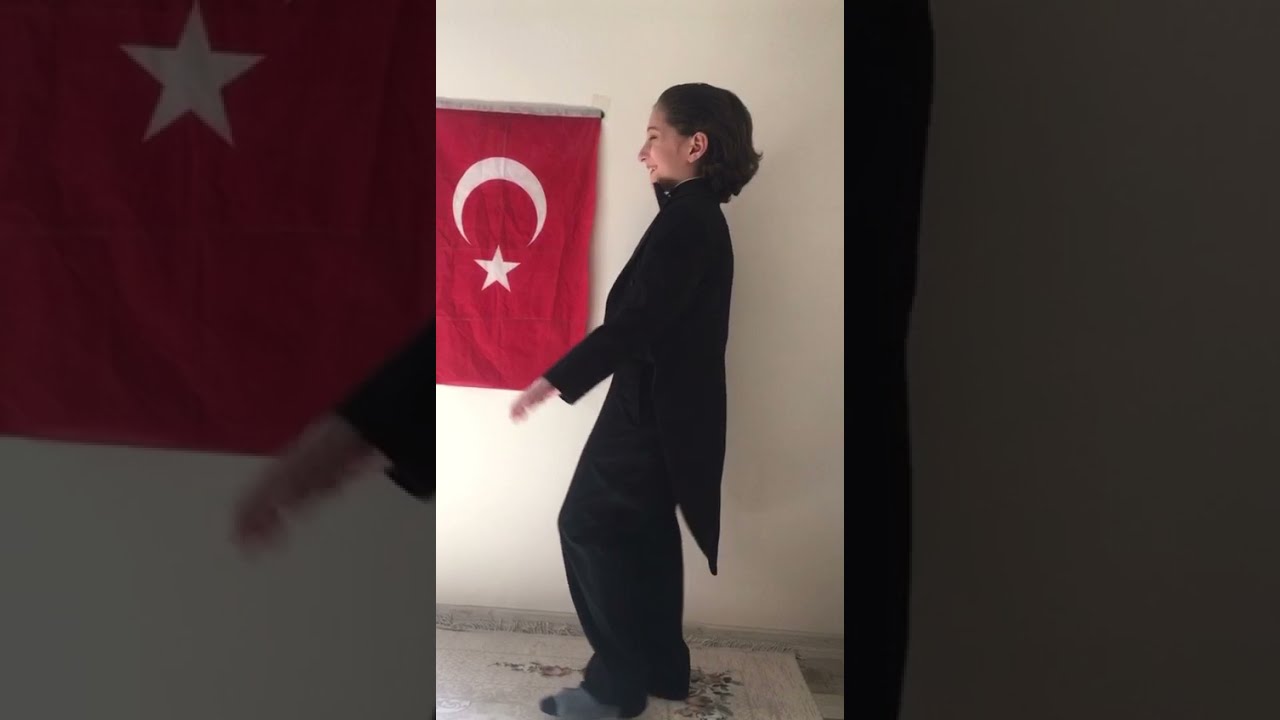The image depicts a woman with short, dark brown hair standing sideways, turned to the left, and smiling. She is dressed entirely in black, including a long-sleeved shirt, pants, and either gray socks or sandals, and a black jacket or cape. Her attire contrasts with the clean, white marble-like floor beneath her feet. Behind her, there is a cream or white-colored wall featuring a red flag with a downward-pointing white crescent moon and a white star, identified as the Turkish flag. The room is split into three vertical sections, with the central section prominently showcasing the woman. The baseboard along the wall appears to be made of stone, and shadows cast by the woman and her surroundings add depth to the scene.